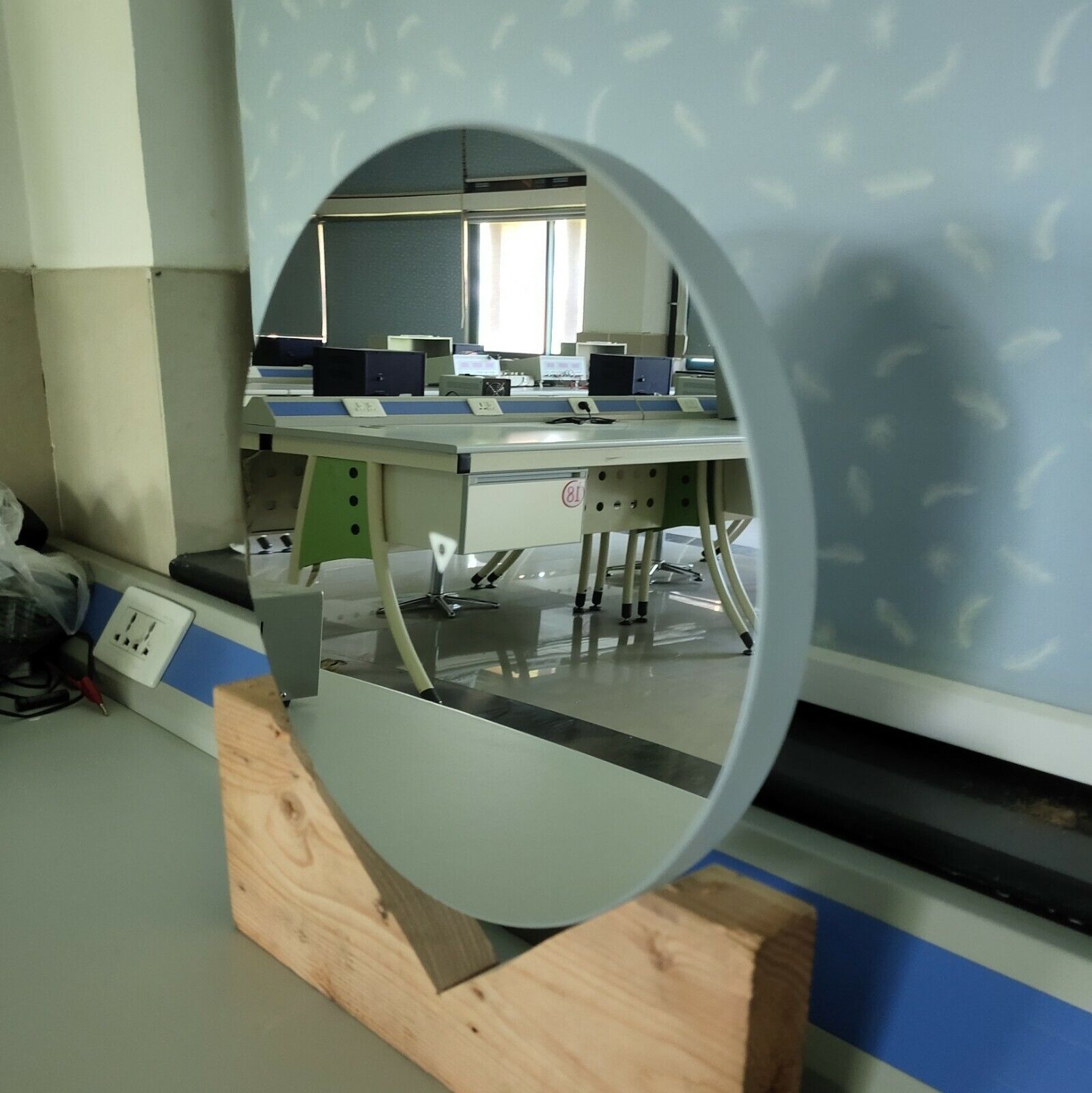The image captures a detailed view inside an office space with a notable blue wall featuring white accents. Central to the scene is a large circular mirror, held by a wooden base with a V-notch cutout. Reflected in the mirror is a bustling office environment, showcasing a variety of desks, both metal and white, with computers, monitors, and various office supplies. The mirror also reveals the presence of black cabinets and a distinctive Bitcoin mining rig, identifiable by its simple rectangular shape and fan. To the left of the mirror, the wall transitions to a two-tone palette, beige on the bottom and cream-colored on the top, accompanied by some red and black wires and an electrical outlet. The floor is white, and the space is adorned with a spectrum of colors including green, tan, black, white, and gray. There is no text visible in the image, which seems to capture a professional, possibly corporate, office setting.